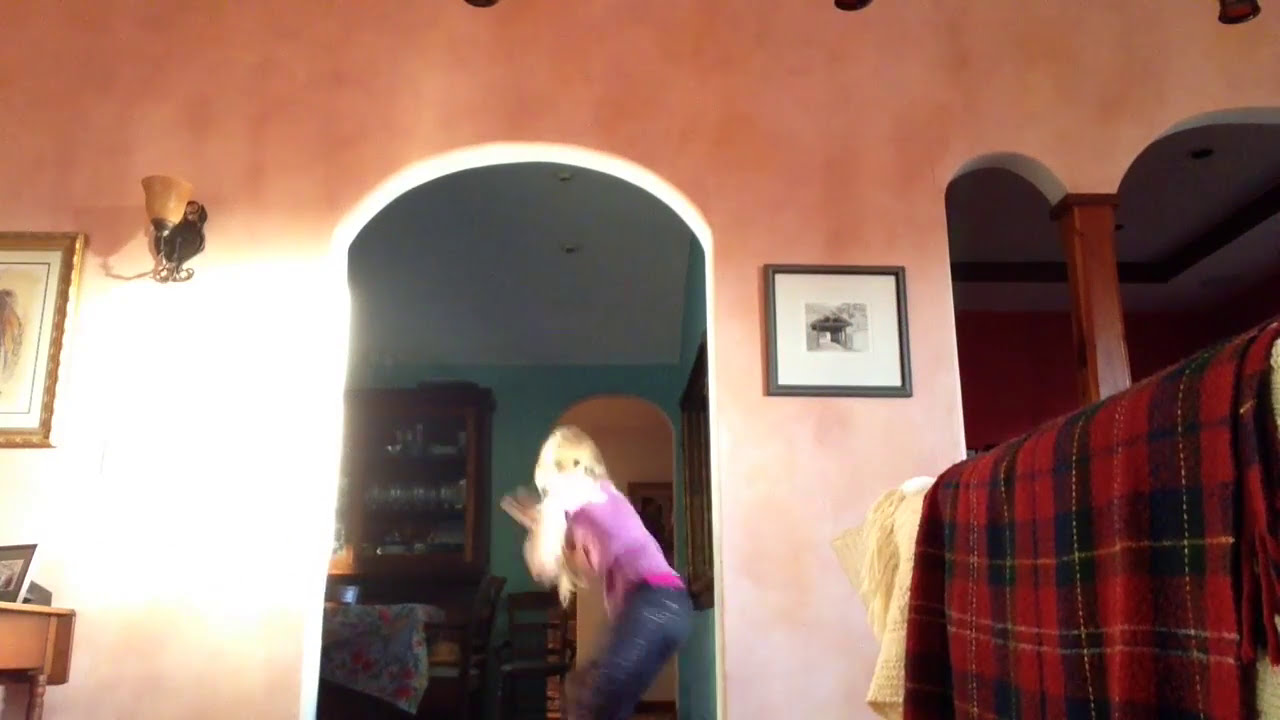The image depicts a cozy interior scene with peach-colored walls and notable rustic elements. Dominating the foreground is the back of a couch adorned with a vibrant, red and black checked blanket. The walls are decorated with various picture frames and a lighting sconce, adding a personal touch to the space. To the right side of the frame, through an arched doorway, we catch a glimpse into another room, identified as a dining area. This room features a large table covered with a colorful tablecloth radiating blues and pinks, surrounded by chairs, and a china cabinet against the back wall. 

In the middle of the doorway stands a woman with blonde hair, wearing a purple shirt and blue jeans. She is somewhat blurred, suggesting movement as if she's turning or shifting position. The bright lighting in the image accentuates her figure as she faces away from the camera. The room she's heading towards has blue-colored walls and a white ceiling, making the transition between spaces distinct yet visually cohesive. The photograph intricately captures the transition between the warm-toned living space and the cooler-toned dining room, creating a harmonious blend of homey and tranquil atmospheres.